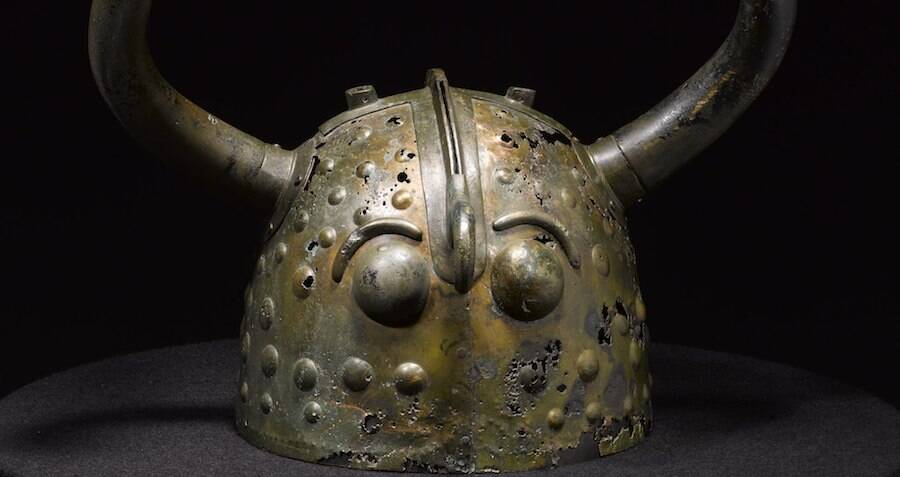In the image, a prominently displayed ancient helmet captures attention against a pitch-black background, with a spotlight illuminating its details. The helmet, likely of Viking origin, features two distinct horns protruding from the sides, each attached with flanged rivets. The metal surface of the helmet is heavily rusted, presenting an earthy gray and green, almost blackened appearance, suggesting significant age and exposure to the elements. The semi-circular dome of the helmet is smooth but marred by chips and cracks, with rivets scattered across its surface. Additional metal casing runs from the top of the helmet down to the center above the nose, featuring a ridge and eyebrow-like grooves. The eye area is marked by smaller domes, adding to the intricate design. The dark setting, combined with the ancient and corroded state of the helmet, evokes an artifact-like relic, possibly more suited for display than actual use.